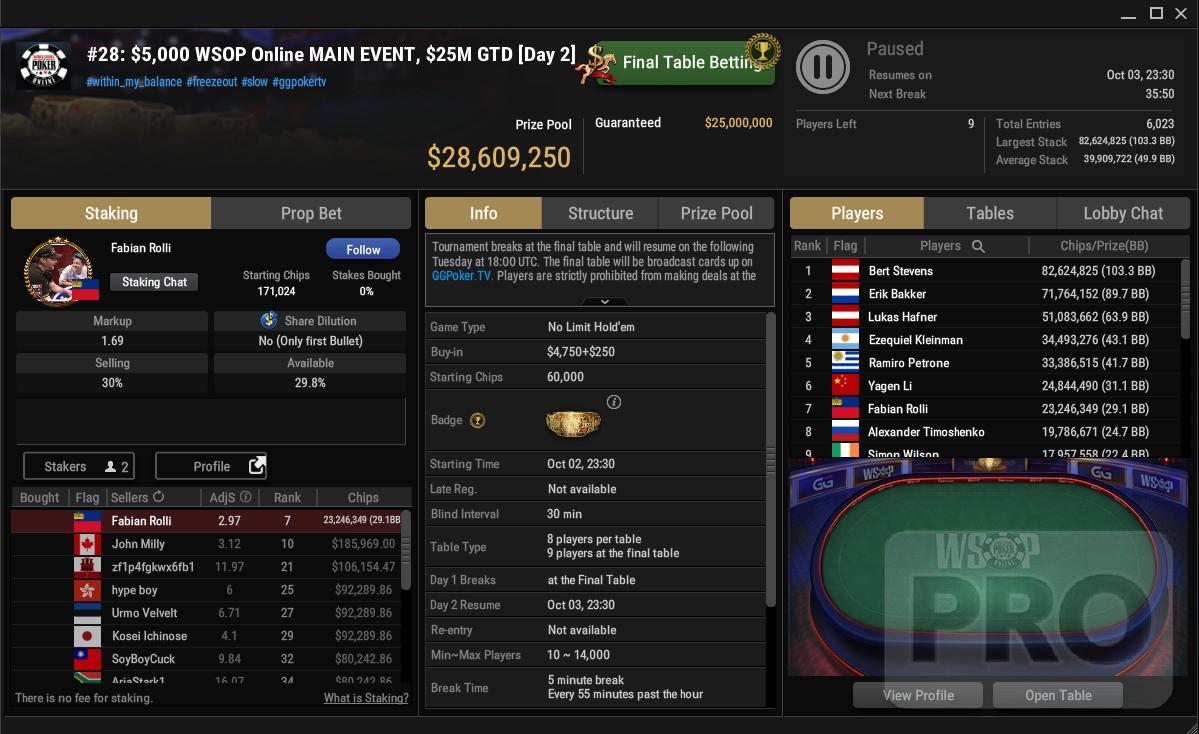In this image of an online poker event, we see detailed information about the "Number 28, $5000 WSOP Online Main Event," highlighted at the top with a prize pool of $25 million guaranteed. The screen is divided into multiple segments. On the upper left, there's a poker chip icon accompanied by event specifics including the No Limit Hold’em game type, the $4,750 + $250 buy-in, and starting chips of 60,000. The central segment reveals extensive tournament details, such as the day two final table betting status, paused status that resumes on the next break, blind intervals of 30 minutes, and that the late registration is closed. It also lists players’ names, their respective country flags, and current chip counts. Leading the board is Burt Stevens with 2,624,825 chips. The bottom right shows a virtual green poker table with a red border, reflecting the game's ongoing nature. The image encapsulates abundant data, including player statistics, prize pool totaling $28,609,250, and the organizational structure of the event, emphasizing the competitive and international aspect of the tournament.